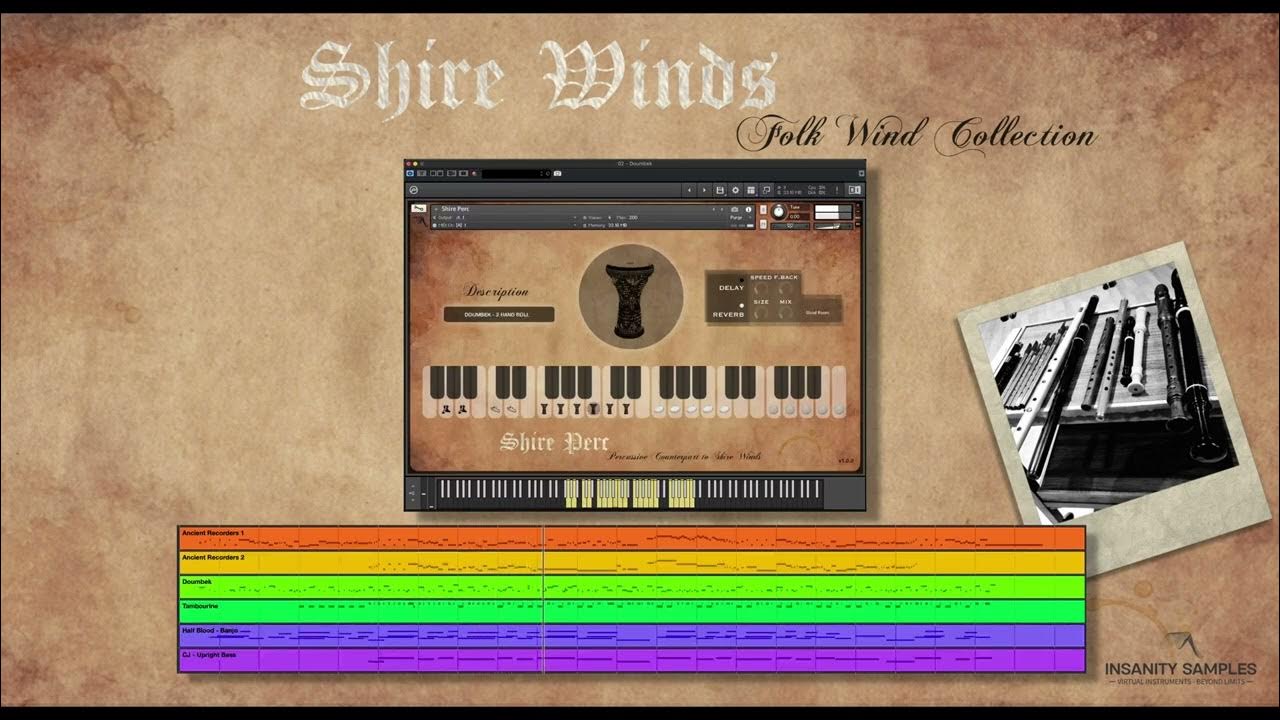The advertisement poster for the "Shire Winds Folkwind Collection" unfolds on an aged tan paper background, reminiscent of parchment. At the top, in elegant white typography followed by italicized black lettering, the title "Shire Winds Folkwind Collection" commands attention. Centrally placed is an evocative image of a computer screen displaying a music program, complete with a small keyboard and a background that mirrors the poster's aged paper texture. To the right, a slightly tilted polaroid photograph features an array of clarinets and wooden musical instruments rendered in black and white. Below, a color-coded time-lapse box with six distinct rows illustrates various graphs, hinting at musical notation. The functionality and aesthetics of the webpage are subtly emphasized by the intricate details. In the bottom right corner, the discreet black text "Insanity Samples" appears, grounding the image with a touch of modern branding. This compelling and detailed layout evokes a sense of nostalgia and musical tradition, seamlessly blending old-world charm with contemporary digital elements.